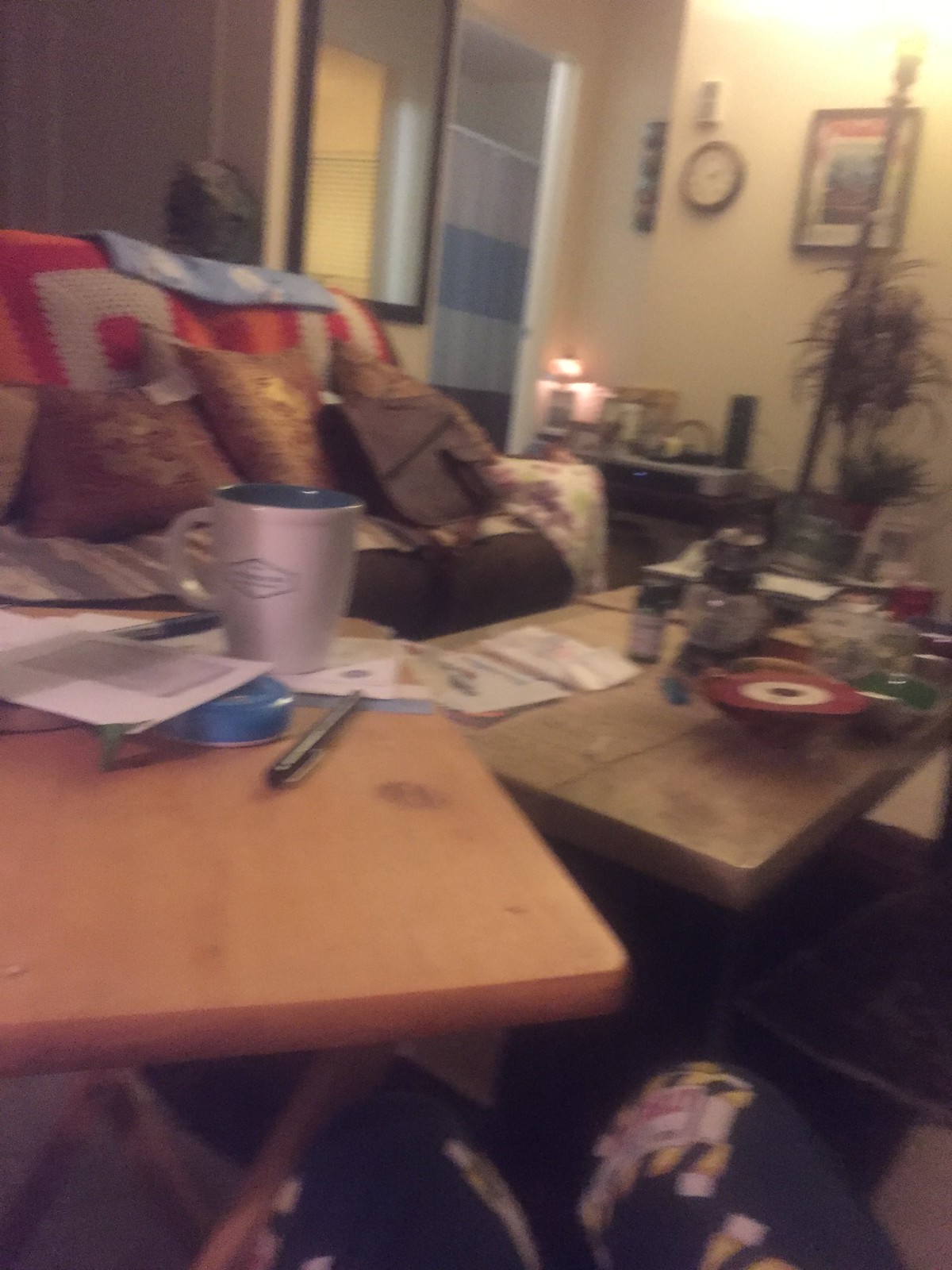An out-of-focus photograph captures a cozy, slightly cluttered living room from the perspective of someone seated in a chair. The person appears to be dressed in casual sweatpants or pajama bottoms adorned with cartoon characters, their legs visible at the bottom of the frame. To the left of the image, a folding table holds a white and blue coffee cup, a pen, a piece of paper, and another small blue object. On the right, a coffee table is strewn with various items including a can of Busch beer, several bowls, and a mix of knick-knacks. A sofa, adorned with pillows, sits against the wall, with a side table displaying a thriving plant. Above the sofa, a lit lamp casts a warm glow, illuminating a clock and a framed photograph on the wall. The room, though a bit messy, exudes a lived-in comfort and could be tidied up swiftly if needed.